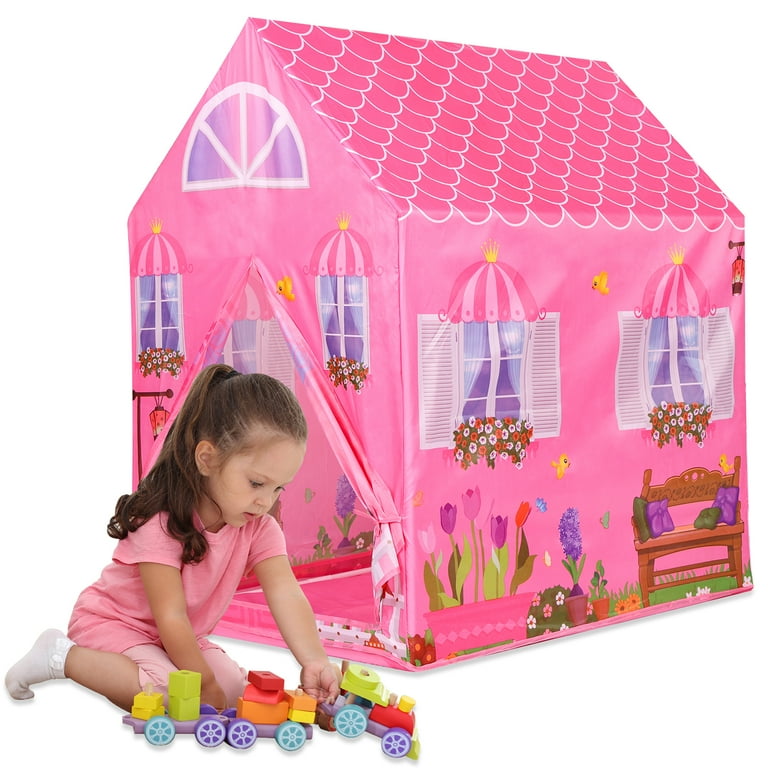In this delightful image, a young girl, approximately four or five years old, is engrossed in assembling a colorful train while sitting on the floor. She has long brown hair neatly tied back in a ponytail, and is dressed in a charming pink outfit consisting of a shirt and shorts. The train she is constructing is vibrantly hued, featuring blue wheels, red blocks, orange blocks, and light green blocks.

In the background, a whimsical pop-up playhouse, resembling a cozy tent, adds to the cheerful atmosphere. The playhouse is predominantly pink with a matching pink roof. Its sides are adorned with artistic details, including windows with white shutters and petite pink curtains above them. Flowers are depicted as growing from windowsills, enhancing the charming look, and imaginary yellow birds are illustrated fluttering around.

One corner of the playhouse showcases tulips, while the opposite side features a quaint bench complete with pillows. The entrance of the tent is open and tied back, revealing a pink interior floor. Above the entrance, another window is positioned, flanked by two more windows below, each framed with similar details of flowers on the sill and pink curtain tops.

Overall, the scene captures a moment of innocent play and vibrant imagination.